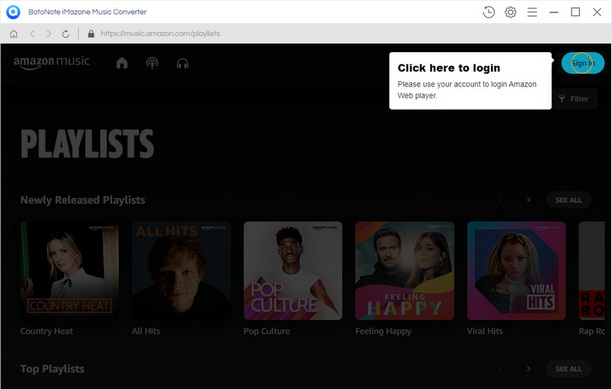The image features a partially obscured music converter interface, presumably by a brand starting with "Bo", though the full name isn't visible. The prominent blue logo includes a "Click here to log in" prompt in bold letters. The interface instructs users to see their account details to log in to the Amazon Web Player. A "Sign In" button is clearly displayed, highlighted within a teal circle. The rest of the interface is blacked out except for the word "playlist," though no specific playlist details are readable.